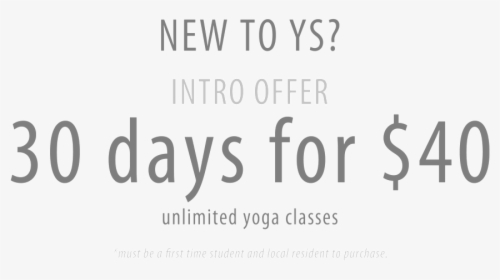A possible advertisement or banner ad features a clean, minimalist design set against a completely white background, blending slightly into an off-white horizontal rectangle. At the top, in a dark gray font, the text reads, "New to YS?" Below that, in a lighter gray, it says, "Intro Offer." The most prominent text, in the darkest gray and largest font, announces, "30 Days for $40." Here, "$40" is displayed with the dollar sign to the left of the number. Just below this, in smaller dark gray text, it states, "Unlimited Yoga Classes." At the very bottom, in extremely light gray and very small print, there is a disclaimer: "Must be a first-time student and local resident to purchase."